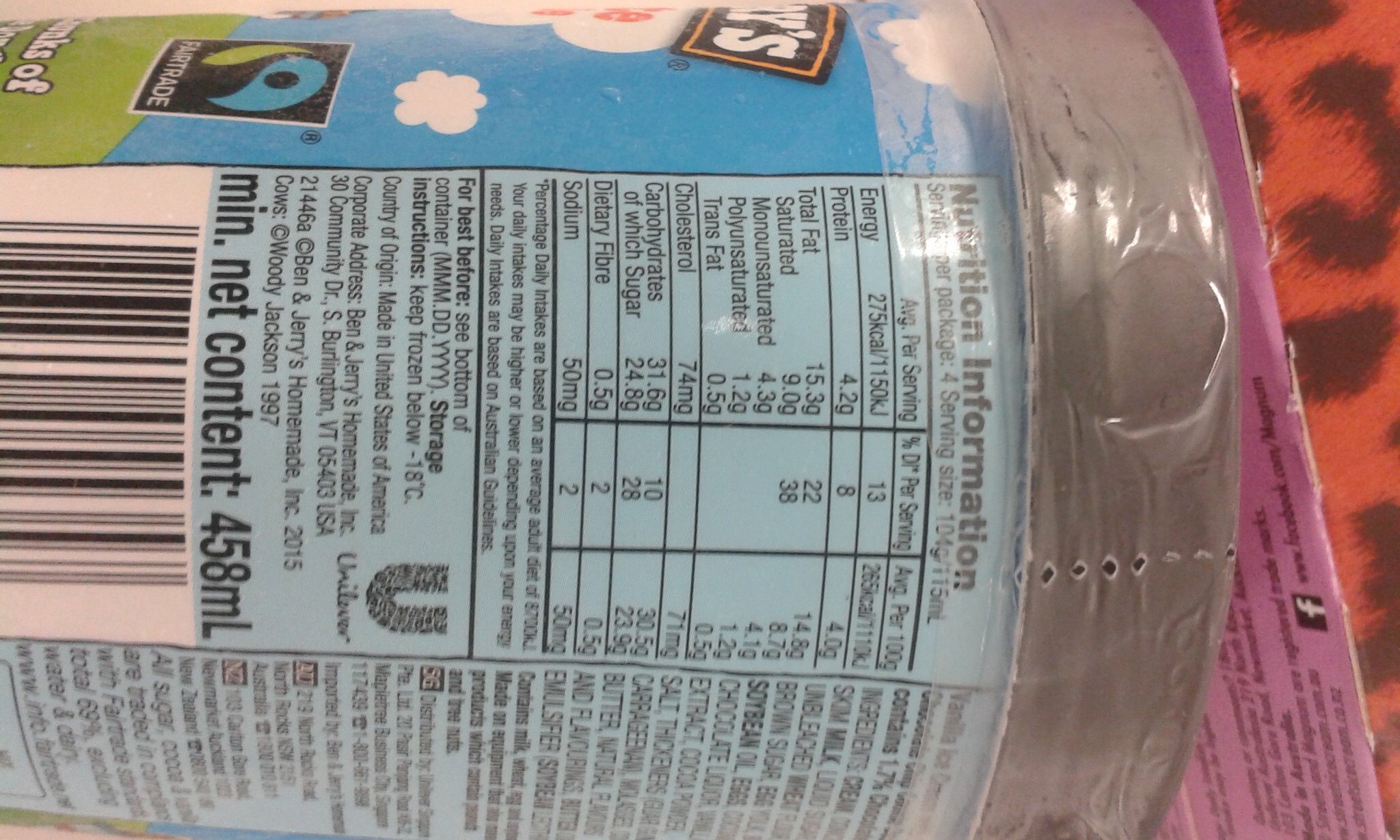This image captures a close-up view of a pint of Ben & Jerry's ice cream laid on its side, prominently featuring the nutrition label at the center. The tub has a distinctive blue and green landscape design with the Ben & Jerry's logo partially visible, along with a Fair Trade logo, both on the side. The lid is brown and cylinder-shaped, still sealed with its original plastic, showcasing perforations for opening. Nutritional details include a serving size of four servings per package with values like 275 kcal energy, 4.2 grams protein, 15.3 grams total fat, of which 9 grams are saturated. It also lists monounsaturated, polyunsaturated, trans fats, cholesterol (74 mg), carbohydrates (31.6 grams, of which 24.8 grams are sugars), dietary fiber (0.5 grams), and sodium (50 mg) per serving. The barcode, a white rectangle with black strips, is clearly discernible. An expiration date and ingredients list are present but partially obscured by the image angle. The background features a texture that is orange and black-spotted, with a purple piece of cardboard visible, containing writing and a Facebook logo. The net content is specified as 458 milliliters, and fluffy clouds decorate the blue sky at the top of the tub. The container remains sealed, ensuring the freshness of its contents.